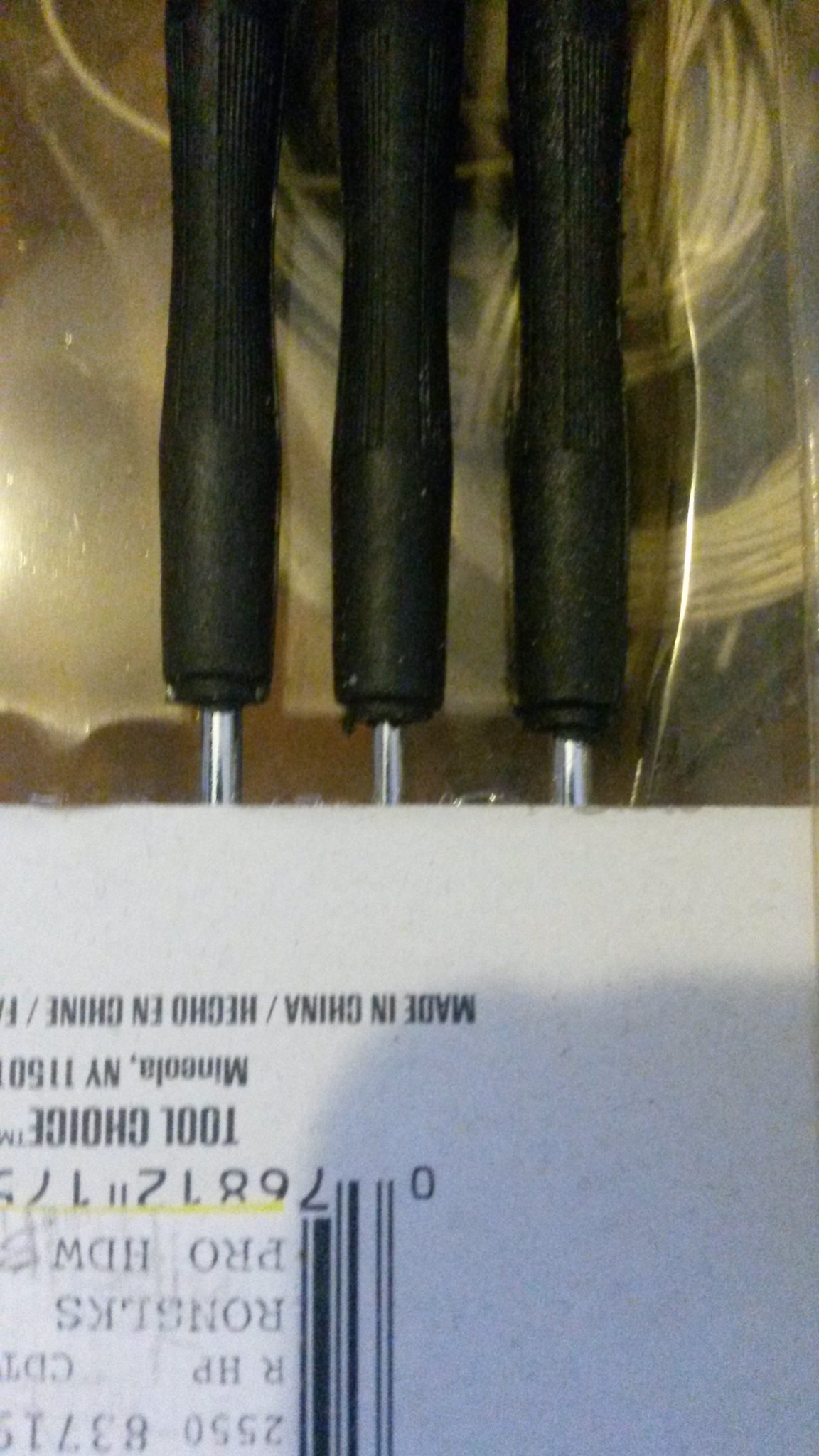This photo depicts a close-up view of an upside-down, partially obscured packaging containing three items with black handles and small, round silver metal extensions at their ends. The items, possibly skewers or very thin screwdrivers, are in a combination of cardboard and plastic packaging. The image also displays a barcode and the text "Made in China" and its Spanish translation "Hecho en China," all visible on the upper portion of the packaging. Despite the poor quality of the image and its awkward angle, it is clear that the items are still encased in their original packaging, with some details difficult to discern due to the image's orientation and clarity.